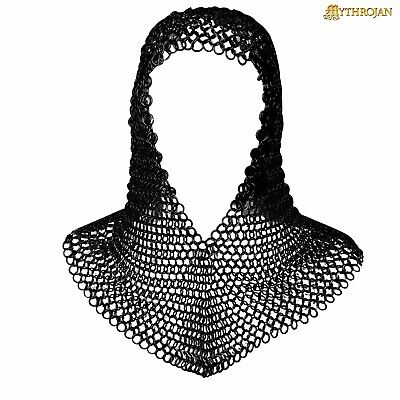The image portrays a medieval-style chain mail hood, intricately crafted with interlinked metal rings that exhibit a fine, mesh-like structure. This piece of armor, commonly worn by knights or soldiers from 1300 to 1600 for protection in battle or jousting competitions, drapes over the head and shoulders, extending down to the middle of the chest. The chain mail's form is sculpted to mimic the human head and shoulders, creating a hood with an opening for the face. The material appears to be gray metallic with a subtle sheen, showcasing the meticulous design of the tiny interlocking circles that give it a flexible yet sturdy texture, akin to scales. The chain mail is set against a stark white background, through which each link can be distinctly seen, and features a yellow logo in the top right corner reading "M-Y-T-H-R-O-J-N, Mithrojan."